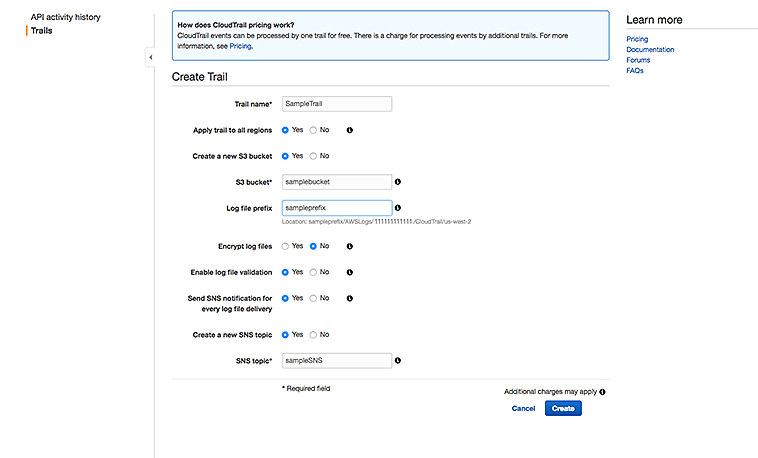**Detailed Caption for Desktop Screenshot:**

The image depicts a screenshot of a desktop interface, specifically an application or web page related to API management and cloud services. The visible content does not reveal the web address, browser type, or operating system in use. 

Starting from the top left, the title "API Activity History" is visible, accompanied by an orange icon that resembles either a pencil or a rectangle, labeled "Trails." Next to it, there's a collapsible arrow, implying the ability to reduce this section to expand the display area.

Central to the interface is a blue-outlined rectangle with a pale blue interior and black text, which asks, "How does CloudTrail Pricing work?" The text explains that CloudTrail events can be processed by one trail for free, but there's a charge for additional trails. A hyperlink labeled "pricing" provides further details.

To the right, there is a "Learn More" section where users can navigate to Pricing, Documentation, Forms, and frequently asked questions (FAQs).

Further down, there is a section labeled "Create Trail," which requires the user to name the trail. In this instance, the trail is named "SampleTrail," written as one word. Users can choose whether to apply the trail to all regions with options "Yes" and "No," with "Yes" currently selected.

The interface offers the option to create a new S3 bucket, toggled between "Yes" and "No," with "Yes" currently selected. Details of the S3 bucket are provided, marked by an asterisk as mandatory, with the bucket name specified as "samplebucket."

The "Log File Prefix" field is filled as "sampleprefix," which includes the location path "sampleprefix/AWSlogo/." The rest of the path is slightly unclear but seems to include numbers and letters, possibly "1515CloudTrailAWS2."

The interface includes options to encrypt log files, enabling log file validation, and sending SNS (Simple Notification Service) notifications for every log file delivery. Currently, encryption is set to "No," log file validation to "Yes," and SNS notification delivery to "Yes." Users can also create a new SNS topic, with the topic name specified as "sampleSNS."

At the very bottom, there is a note stating that fields marked with an asterisk are required and additional charges may apply, with further information available via a hyperlink. Users can finalize their configurations by selecting either "Cancel" or "Create."

Overall, the interface appears to be part of a cloud service platform, likely related to AWS CloudTrail, which tracks user activity and API usage within a cloud environment.